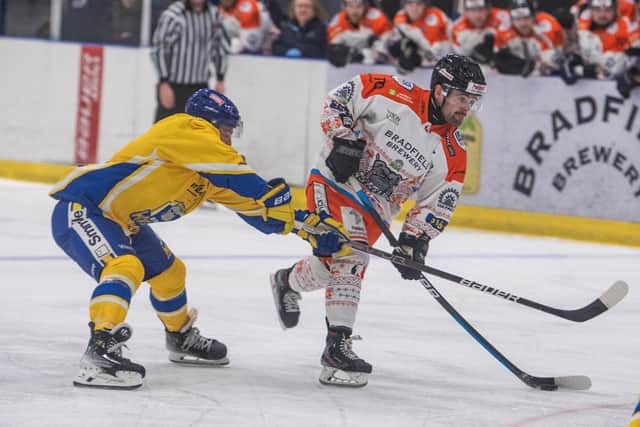The photograph captures an intense moment in an ice hockey game. In the foreground, two players are vying for control of the puck. The player on the left wears a yellow and blue jersey, blue pants, and yellow socks with blue and white stripes above the ankle. His opponent, the player on the right, is dressed in an orange jersey with blue sleeves, orange pants, and a white helmet. Both players are equipped with black gloves and black skates. The player in the orange jersey is shooting the puck with his Bauer stick, which features white tape on the blade, while the yellow and blue player attempts to block the shot with his stick. In the background, a referee, donned in a long-sleeved black and white striped shirt, oversees the action. Leaning over the bench, players from the team in white jerseys with orange shoulders and black helmets watch the game with anticipation. There's a visible board with sponsors and a yellow border stripe, marking the boundary of the rink.